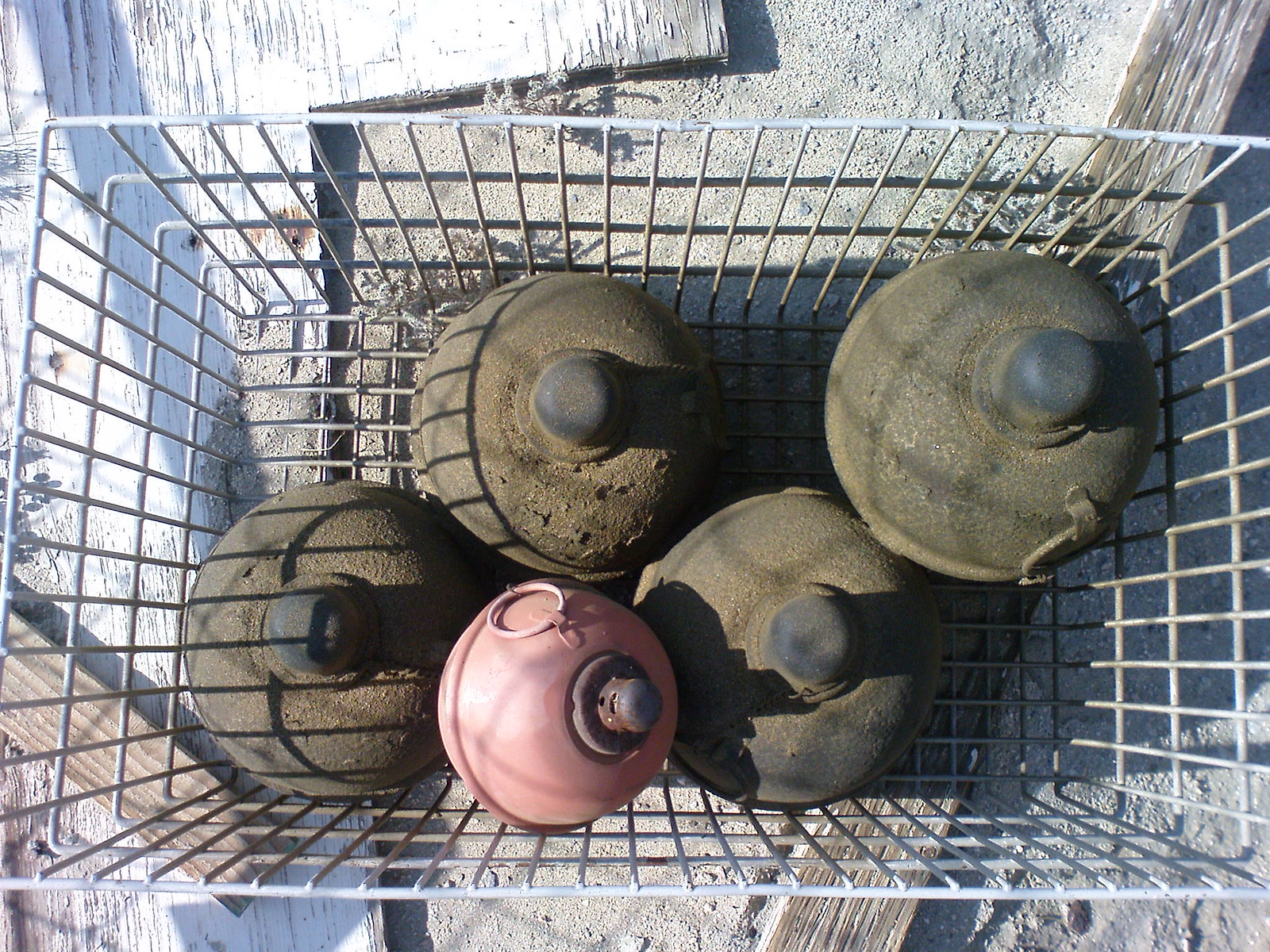The photograph shows a silver wire basket that appears well-weathered with some wires turned brown from exposure. Inside the basket, resting on a layer of gray sand laid atop wooden planks of varying colors, lie five objects that resemble World War II-era artillery. Four of these objects are large, rusted, dirt-covered bombs with circular tops and soldered loops. Their deteriorated state suggests long-term burial or exposure to harsh conditions. In contrast, one smaller, pink object, also featuring a circular top and a loop, stands out due to its relatively smooth surface and lack of rust or severe damage. The entire scene, framed by the basket settled amidst a backdrop of wooden boards and sparse weeds, exudes an air of historical detritus.